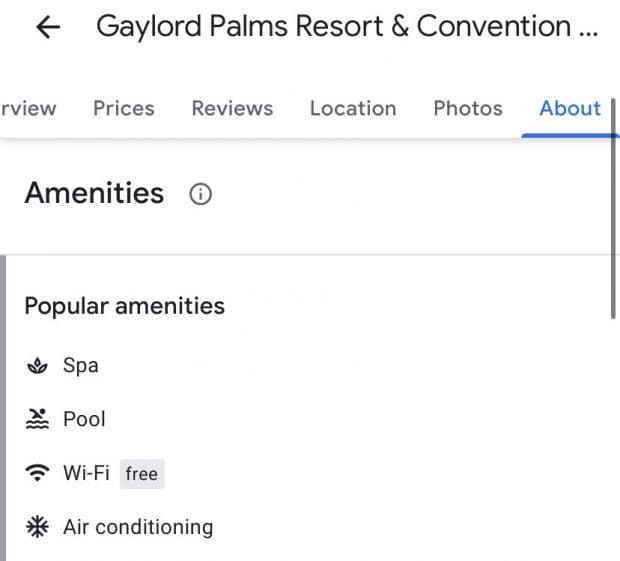The image displays a section of a website with a white background. At the top left, there is a black arrow pointing to the left. Next to the arrow, the text "Gaylord Palms Resort & Convention..." is prominently featured with capitalized initials (G, P, R, C) and an ampersand symbol representing "and." Directly below, partially visible text starts with "this is RVI," using lowercase letters, likely part of the word "review."

Further down, the website features tabs for "prices," "reviews," "location," "photos," and "about." Of these, the "about" tab is highlighted in blue text and underlined with a blue line. A thin divider line separates these tabs from the content below.

Beneath this divider, the bold heading "Amenities" starts with a capital A. Right next to it is a small, grey-outlined circle containing a lowercase, grey "i" (likely an information icon). Another thin line appears below, followed by the heading "Popular Amenities," with a capital P.

Under "Popular Amenities," various icons represent different features: a lotus leaf symbol for the spa, a swimmer icon for the pool, a Wi-Fi signal icon labeled "free" for complimentary wireless internet, and a snowflake icon for air conditioning.